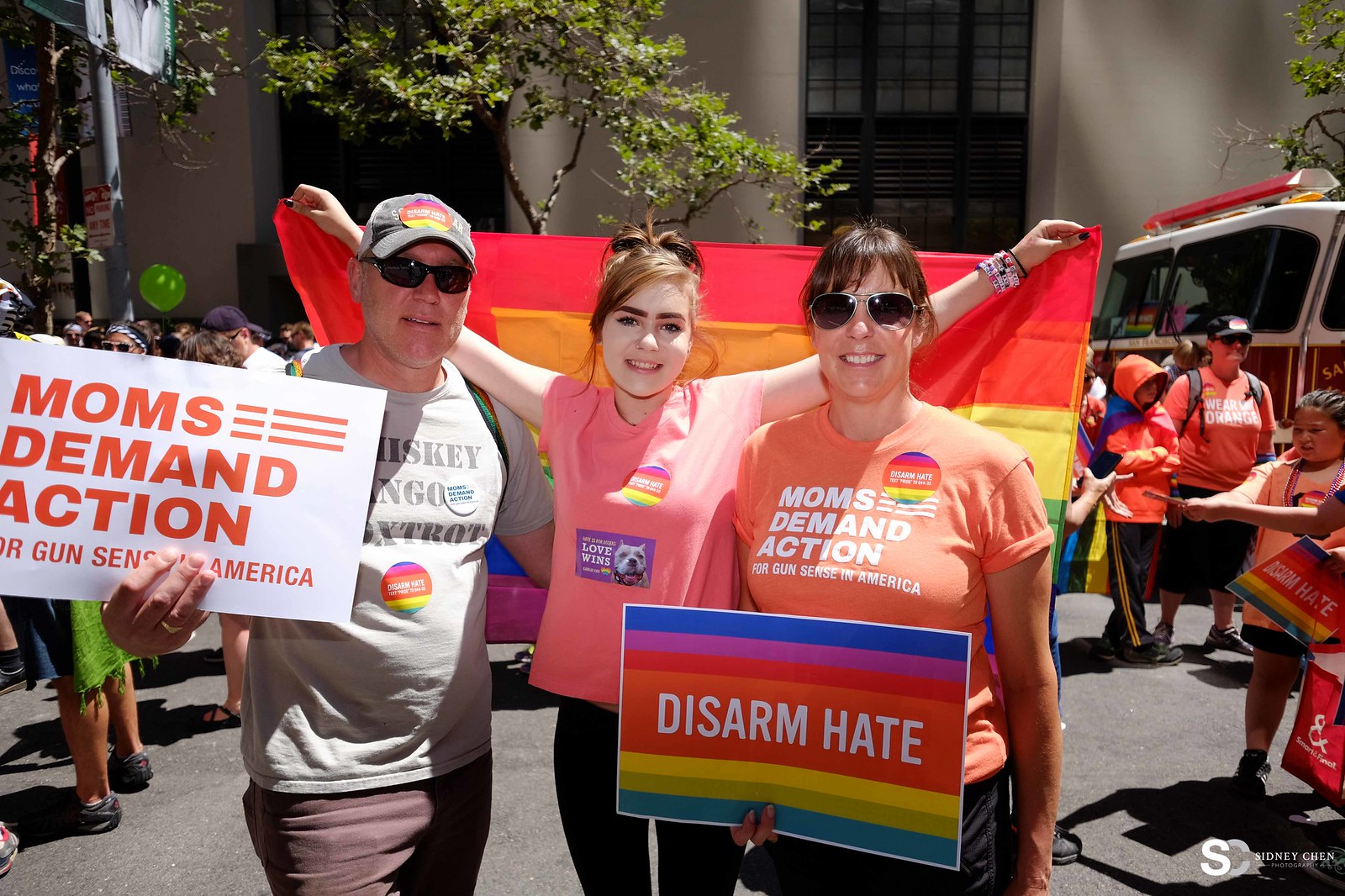The photograph captures an outdoor protest during the day, featuring a group advocating for gun control in the United States. At the center of the image stand three committed activists: a man on the left, an older woman on the right, and a younger woman between them. The man, with gray hair and a dark baseball cap adorned with a rainbow sticker, holds up a white sign that says "Moms Demand Action for Gun Sense in America." The woman on the right, wearing a salmon-colored shirt with the same text, carries a sign with horizontal rainbow stripes that reads "Disarm Hate." Between them, the younger woman, approximately 17 years old and wearing a pink t-shirt with a rainbow "Disarm Hate" sticker and another sticker that says "Love Wins," stands with her arms outstretched, holding a rainbow flag. All three individuals wear sunglasses and embody a spirit of unity and determination. Behind them is a lively street scene with other protesters, many in similar-colored shirts, a visible fire truck in the top right corner, and a building in the backdrop, contributing to the bustling protest atmosphere.